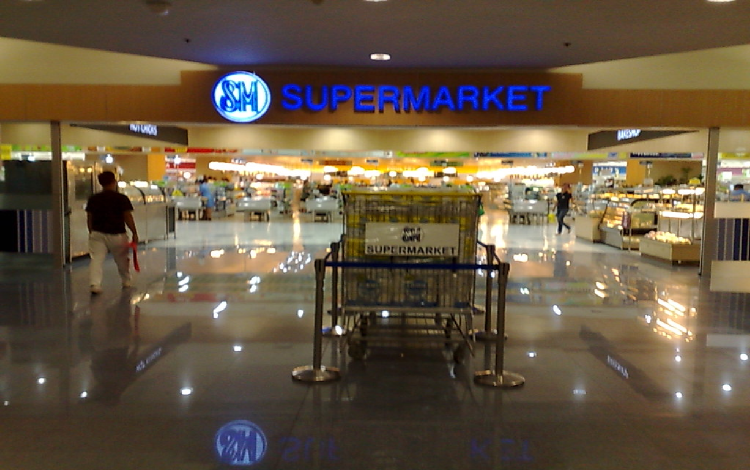The image depicts the entrance of an SM Supermarket, identifiable by the prominent logo at the top center of the entrance. The logo features a white oval with a blue edge, displaying the letters "SM" in blue, and the word "Supermarket" to its right. Below this sign, a large shopping cart is centrally positioned, surrounded by silver cylindrical poles sectioning it off with a line divider. The cart itself has a sign with the supermarket's name in black, all-caps letters on a white background. The supermarket interior starts with light brown tiles which transition into white tiles further inside, presenting a clean appearance. 

On the left side of the image, a man in a short-sleeved black shirt and khaki pants is walking towards the entrance, holding a red item in his hand. In contrast, on the right side, a woman in jeans and a black short-sleeved shirt is walking towards the camera, seemingly leaving the store. The background features blurred items and store departments, notably a bakery section near the woman. The image gives a detailed view of both the exterior signage and some interior elements of the SM Supermarket, highlighting its clean and organized layout.